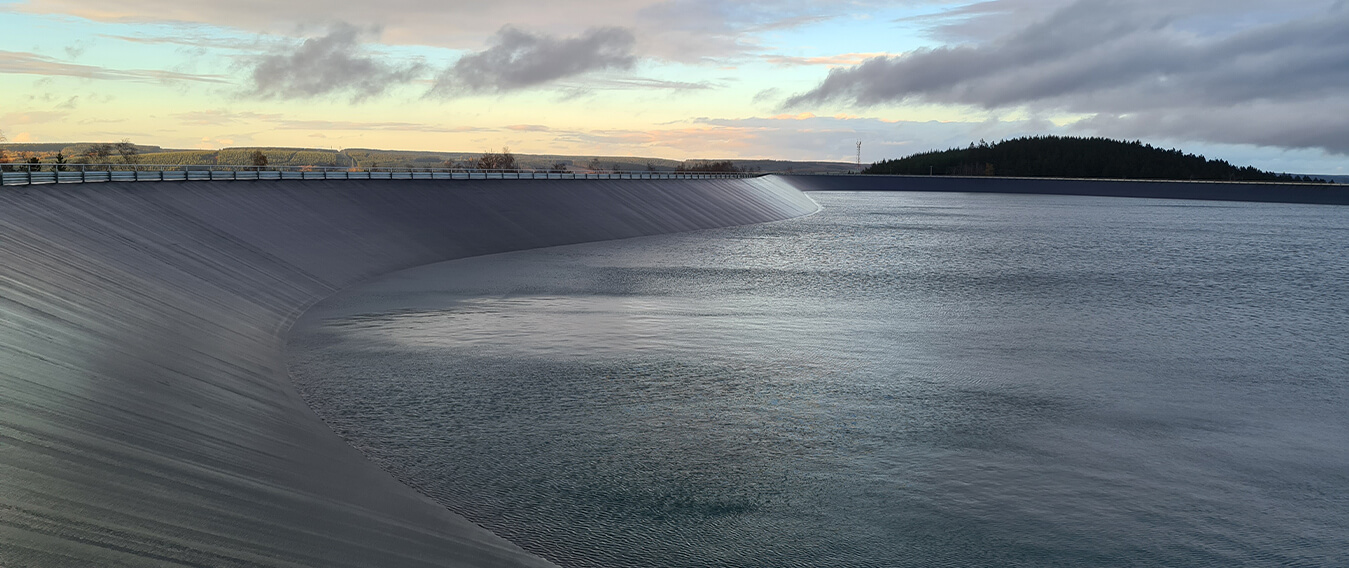The photograph showcases an outdoor scene featuring a man-made reservoir, bordered by a concrete barrier that supports a roadway. The glistening water occupies the left portion of the image, creating a vivid contrast with the slanted concrete structure on the right. This barrier extends upwards at a slight slope, culminating in a guardrail-enclosed road that winds across the top edge of the photograph. In the background, the serene sky is painted with hues of blue and pink, decorated by wisps of clouds, indicative of either sunrise or sunset. The distant horizon is adorned with a tree-lined hill, adding depth and natural beauty to the composition.